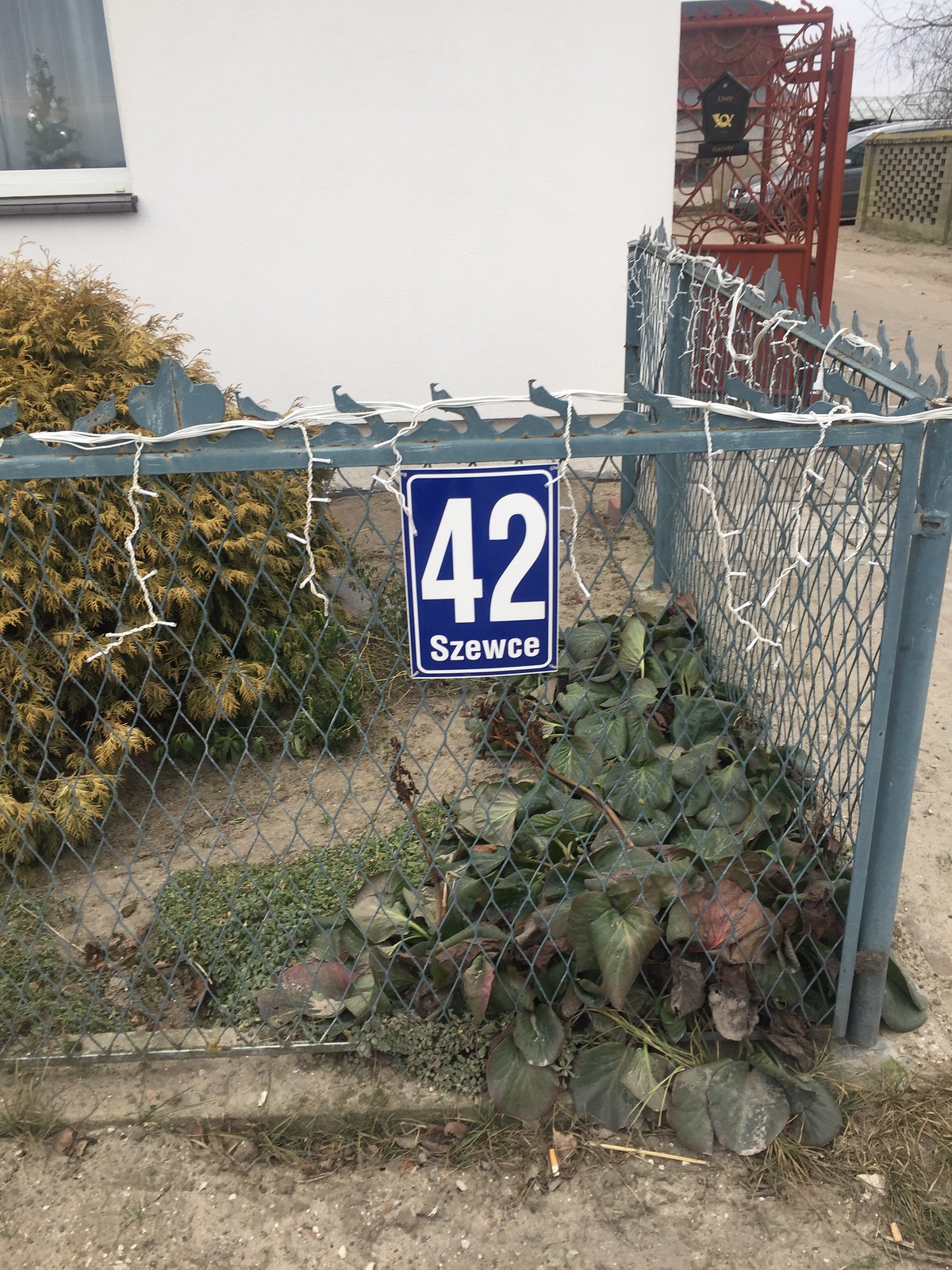This detailed photograph captures a side view of a white house with a yard enclosed by a three-foot high chain link fence adorned with spikes at the top. Interwoven through the spikes are white Christmas lights, giving a festive touch. Centered on the gray metal fence is a navy blue square sign with large white numerals displaying '42' and the Polish word 'Szewce' spelled out in white letters. In the foreground, lush greenery is evident with overgrown leaves and various plants crowding near the bottom of the fence, particularly to the left. Additionally, a bush exhibiting yellowish, orangey, and brown hues is prominently visible. In the background of the yard, a small decorative Christmas tree is seen through a window in the upper left corner of the house. To the upper right, a porch enclosed by a striking red metal gate is discernible. The overall setting suggests a quaint, slightly overgrown garden scene adjacent to a cozy, festively adorned home.